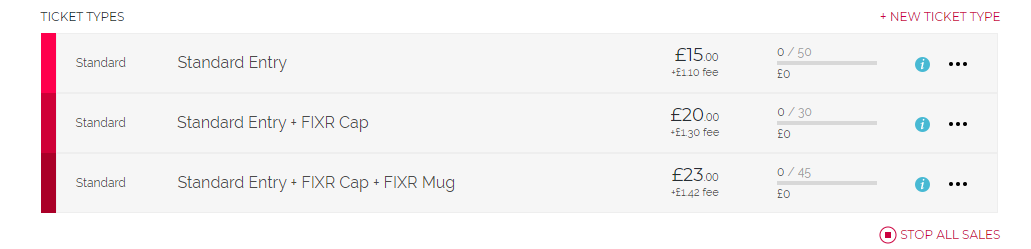The image from the website appears to be part of a ticket-selling platform named FIXR. The interface is specifically designed for sellers. The main section of the interface is divided into three columns, with the leftmost column labeled "Ticket Types." On the far right, there's a red button labeled "Plus New Ticket Type," allowing the seller to add additional types of tickets.

The "Ticket Types" column lists three different options, all categorized under "Standard":

1. **Standard Entry**: 
   - Price: £15.00
   - Available Tickets: 50 (denoted with 0/50 above the price, indicating none have been sold yet)
   - Earnings: £0.00

2. **Standard Entry plus FIXR Cap**:
   - Price: £20.00
   - Fee: £1.30
   - Available Tickets: 30 (denoted with 0/30 above the price, indicating none have been sold yet)
   - Earnings: £0.00

3. **Standard Entry plus FIXR Cap plus FIXR Mug**:
   - Price: £23.00
   - Fee: £1.42
   - Available Tickets: 45 (denoted with 0/45 above the price, indicating none have been sold yet)
   - Earnings: £0.00

At the bottom right of the interface, there is a link titled "Stop All Sales," which presumably allows the seller to halt all ticket transactions.

The detailed breakdown gives a clear understanding of the types of tickets available for sale, their prices, associated fees, and the current sales status.